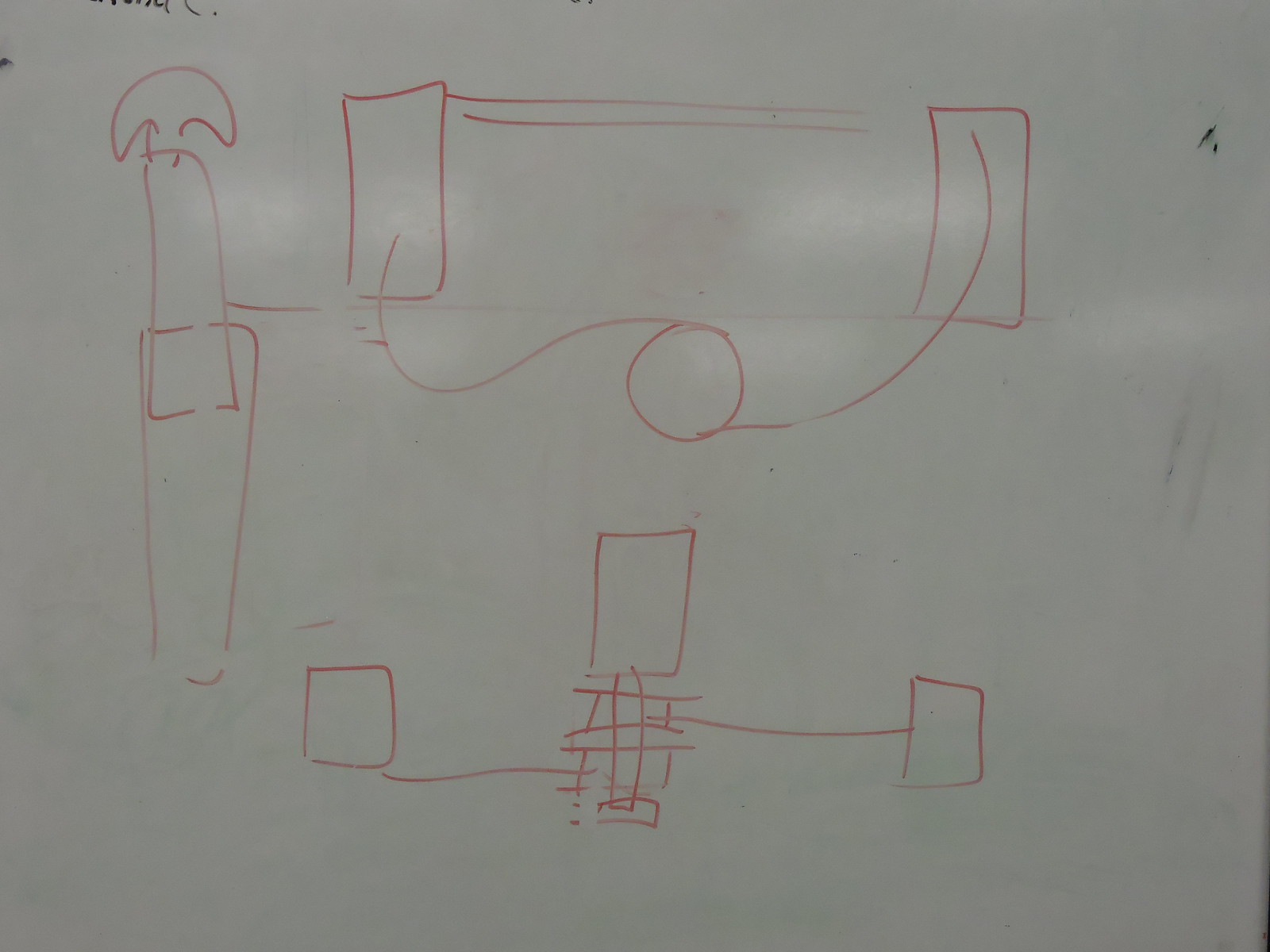This photograph captures a detailed drawing on a whiteboard, rendered in a rust-colored red marker. The composition is intricate, featuring various geometric shapes and lines. At the bottom of the board, there are three horizontally aligned rectangles, connected by lines: one on the right, one on the left, and one in the center. Multiple lines link the central lower rectangle to a smaller rectangle situated directly above it, forming a network-like structure. Below the smaller central rectangle, a shape resembling a Chinese pagoda is depicted.

In the upper section of the image, two vertically standing rectangles (longer sides on the top and bottom) are drawn. Two horizontal lines emerge from the left rectangle, extending towards the right rectangle but stopping before reaching it. The lower horizontal line does not touch either rectangle. Centrally placed at the top is a circle, from which a line extends to the left rectangle and right through to the top of the right rectangle.

On the left side of the image, a nearly complete rectangle intersects with another rectangle about 20% from the top. Above this intersection, a half-moon shape with its points directed towards the rectangle is illustrated. Additionally, the right side of the image shows some black smudges, possibly remnants of previous drawings or text.